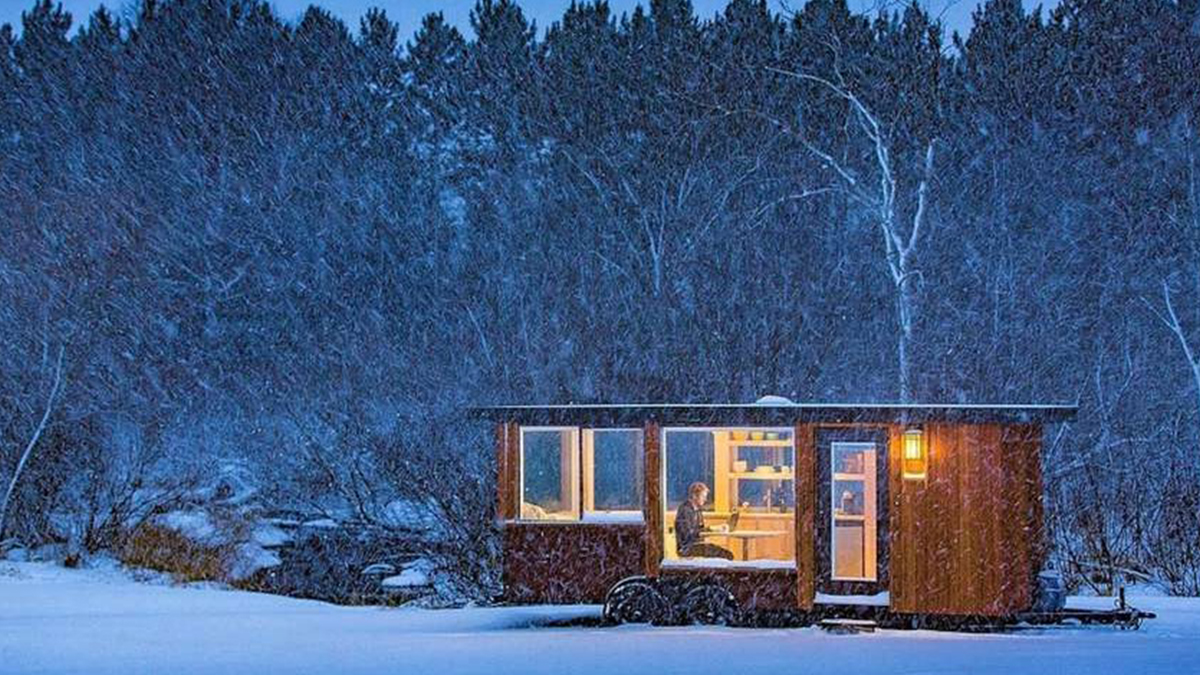The image captures a multi-colored, horizontally rectangular artwork depicting a serene winter night outdoors. Dominated by a deep blue nighttime sky, the background features a dense forest with both pine and bare trees. Snow blankets the ground, accentuated by a thick snowfall, creating a peaceful, cold atmosphere. In the lower left corner, stacks of firewood are visible, adding a rustic touch. The main focus is a brown wooden trailer with multiple windows, illuminated warmly from within. Attached to the trailer are two black tires, emphasizing its mobility. Inside the trailer, a young man is seated at a table, engrossed in his computer, with shelves of plates and bowls visible behind him. He appears isolated and cozy amidst the storm, surrounded by the natural beauty and tranquility of the snowy woods.